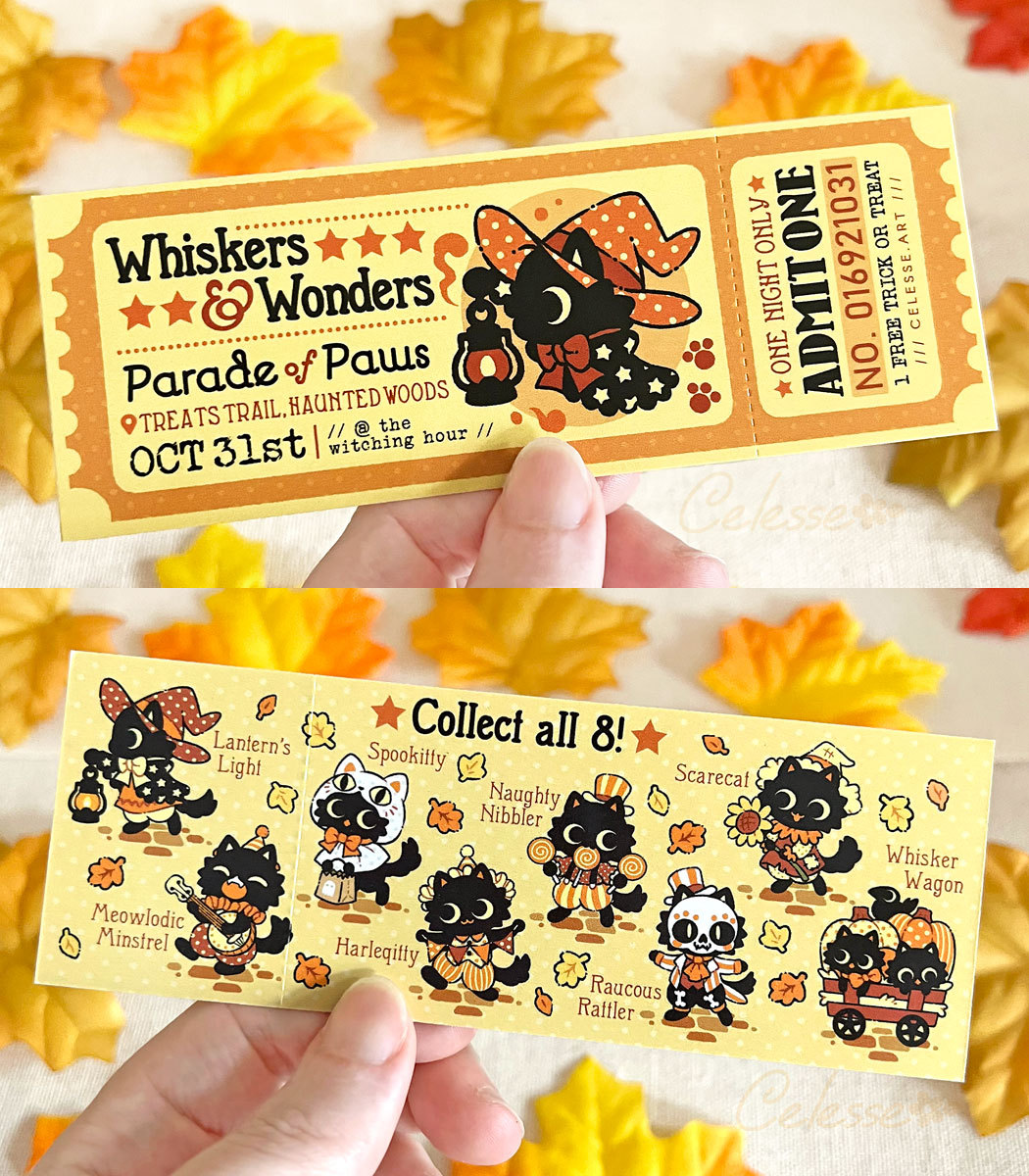The image features two beautifully crafted event tickets, each held by a hand, with a backdrop of yellow and orange autumn leaves that evoke a cozy, Halloween spirit. The top ticket promotes a whimsical Halloween event titled "Whiskers and Wonders: Parade of Paws, Treats Trail, Haunted Woods" set for October 31st at the witching hour. It also boasts the tagline "One Night Only" and "Admit One," with an admission number 016921031 and an offer for "one free trick or treat" from celeste.art. The design is enhanced by a charming illustration of a black cat wearing a polka-dot witch's hat and holding a lantern.

Overlaying the first image, the second ticket invites the viewer to "Collect All Eight," showcasing different versions of the same adorable black cat in thematic costumes: "Lantern's Light" with a witch's hat and lantern, "Meowdic Minstrel" playing a banjo, "Spooky Kitty" dressed as a ghost, "Harlequitty" resembling a clown, "Naughty Nibbler" holding large lollipops, "Raucous Rattler" donning a Day of the Dead skull mask, "Scare Cat" as a scarecrow, and "Whisker Wagon" featuring two cats in a wagon with a crow atop. The tickets merge artistic charm with festive vibes, making them perfect collector's items that one might proudly share on Pinterest or purchase on Etsy.